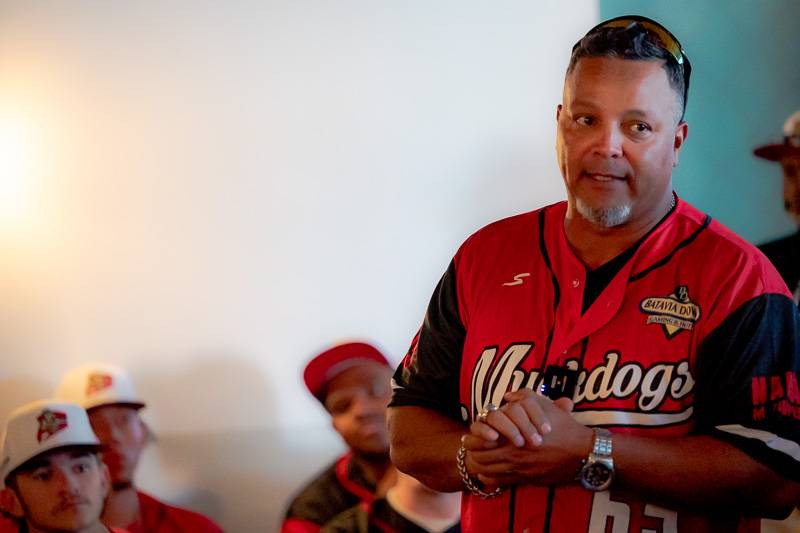This photograph, taken at Eli Fish, captures the introduction of the 2023 Muckdogs team to their fans. In the foreground, a man stands on the right, sporting a Muckdogs baseball jersey that is predominantly red with black sleeves and white lettering spelling out "Muckdogs." His jersey bears the number 63, partially concealed as he holds his hands across his chest. He has a gray beard, brown hair, and his sunglasses are pushed up over his head. He wears a gold bracelet and a silver watch. Behind him, the background features an off-white wall with out-of-focus fans, all donning various baseball caps with white fronts and black bills, attentively listening to the introductions. Another man, also in a Muckdogs jersey and a white hat, appears slightly out of focus to his left. The overall scene vividly showcases the excitement and engagement of both team members and fans at this celebratory event.